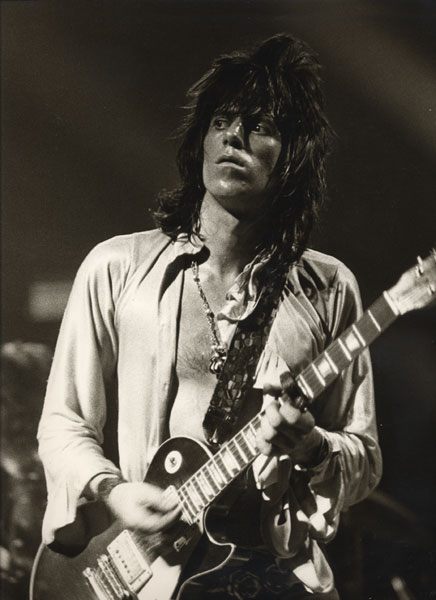In this black-and-white photo, a young Keith Richards is captured mid-performance with his guitar. The image, though monochromatic, has subtle brownish tones, giving it a nostalgic feel. Keith, adorned in a light-colored, loose and flowy button-up collared shirt left open to reveal his chest and a pendant necklace, stands out with his pronounced cheekbones, strong nose, and intense dark eyes. His long, layered black hair, styled into a mullet with bangs, cascades to his shoulders. Keith's serious expression is directed to his right, while both hands grip the guitar, secured by a strap slung across his chest. A faint, blurred background with varying shades of brown and gray frames this iconic moment, highlighting the rock and roll legend immersed in his music. Additionally, a sashy scarf can be seen hanging from his left shoulder, adding an extra touch of rockstar flair to his ensemble.